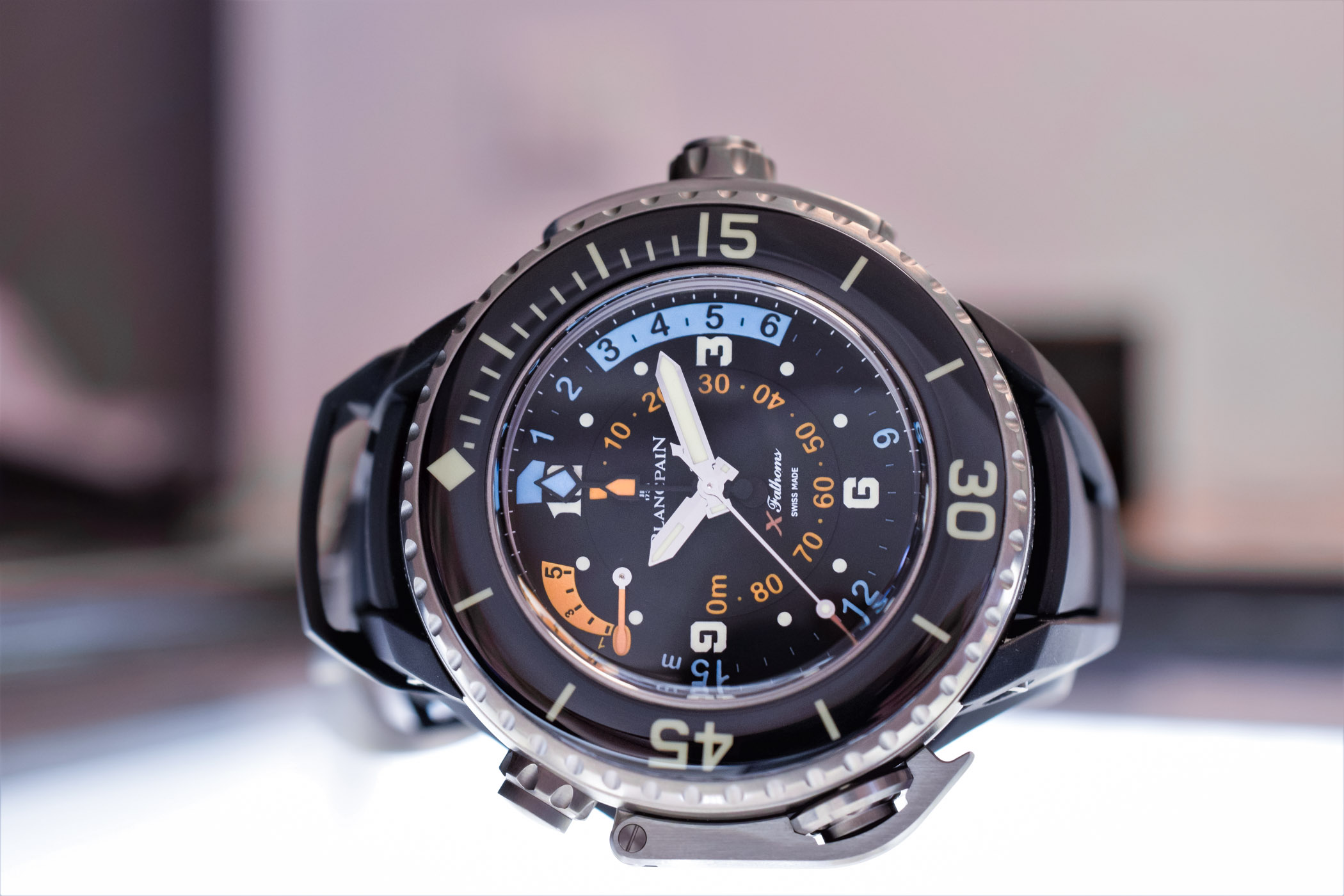This close-up photograph focuses on an intricately detailed watch face, set against an off-white, blurred background. The watch, lying on its side, is held by a bright white stand that appears to be illuminated. The watch itself is predominantly silver, including the barely visible band and the adjustment knobs on the side.

The central face of the watch is marked by contrasting features: white hour, minute, and second hands prominently display the time of 10:12. Surrounding these hands, the inner ring features gold-ish white numbers with small blue increments that resemble a mileage gauge. Additionally, there are orange numbers arranged in a circular pattern from 10 to 80. The dial includes the letters "G" and "OEM," adding to its unique design elements. 

Encircling the core, the outer rim acts almost like a compass, marked with large numbers at intervals of 15, 30, and 45, interspersed with lines and a star symbol. This ring is bordered by a silver colored edge, enhancing its lustrous appearance. The detailed design not only showcases the time but also an array of additional functional elements, making it both a visual and practical centerpiece.